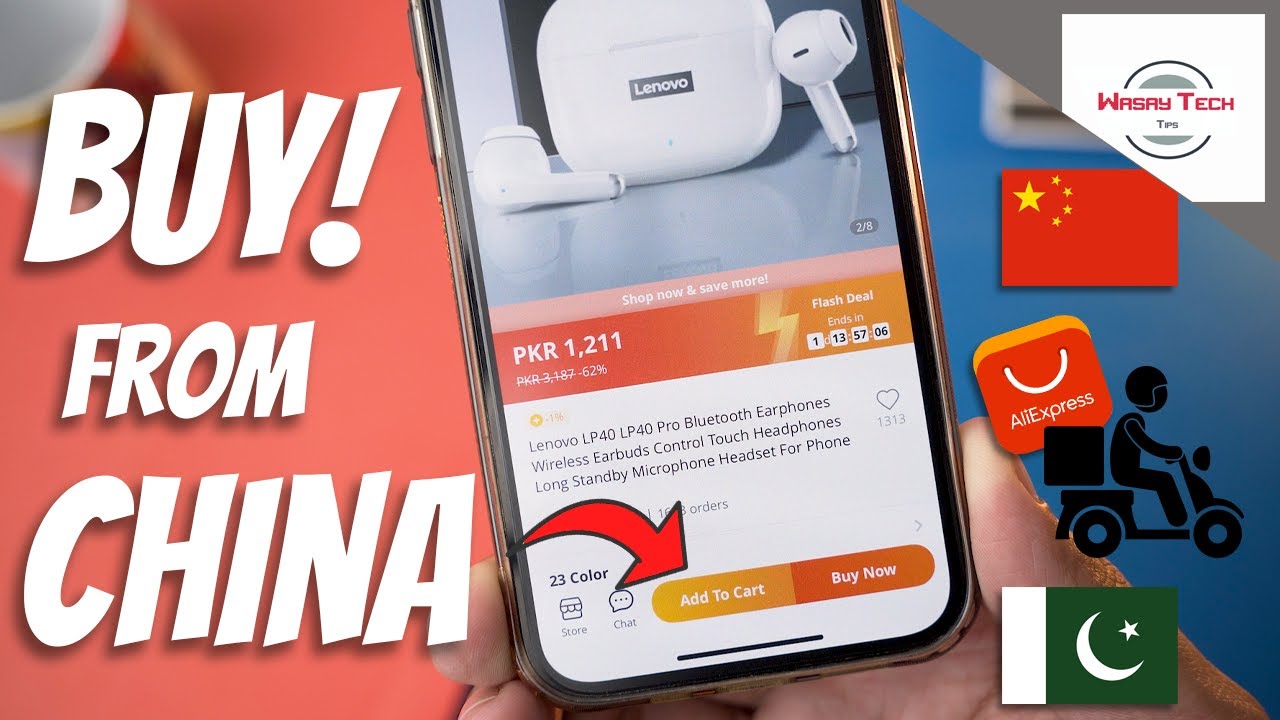This image is a vibrant, graphical advertisement featuring a photograph overlaid with text and various icons. At the center of the image, a person is holding up a mobile phone towards the camera, displaying a shopping app on the screen. The app showcases a set of wireless earbuds, accompanied by product details and options to "Add to Cart" or "Buy it Now." 

Dominating the left side of the image, large white text reads "Buy! from China," with an arrow pointing towards the "Add to Cart" button on the phone screen. Surrounding this text are several graphical icons and elements. 

To the left of the phone screen, a white box labeled "Wasatec Tips" is prominently displayed. Adjacent to this, a red flag featuring one large yellow star and four smaller yellow stars sits in the top-left corner, symbolizing China. Below this flag, an Aliexpress icon depicted as a red bag is present, implying the shopping platform. Additionally, there is a black icon of a person riding a scooter with a delivery box, signifying fast delivery services. Another national flag, green and white with a crescent moon and a small star, likely representing the flag of Pakistan, is also featured, indicating international shipping or a target market.

This advertisement is crafted to attract attention and stimulate shopping interest by highlighting the ease of purchasing products from China through a popular online shopping app.